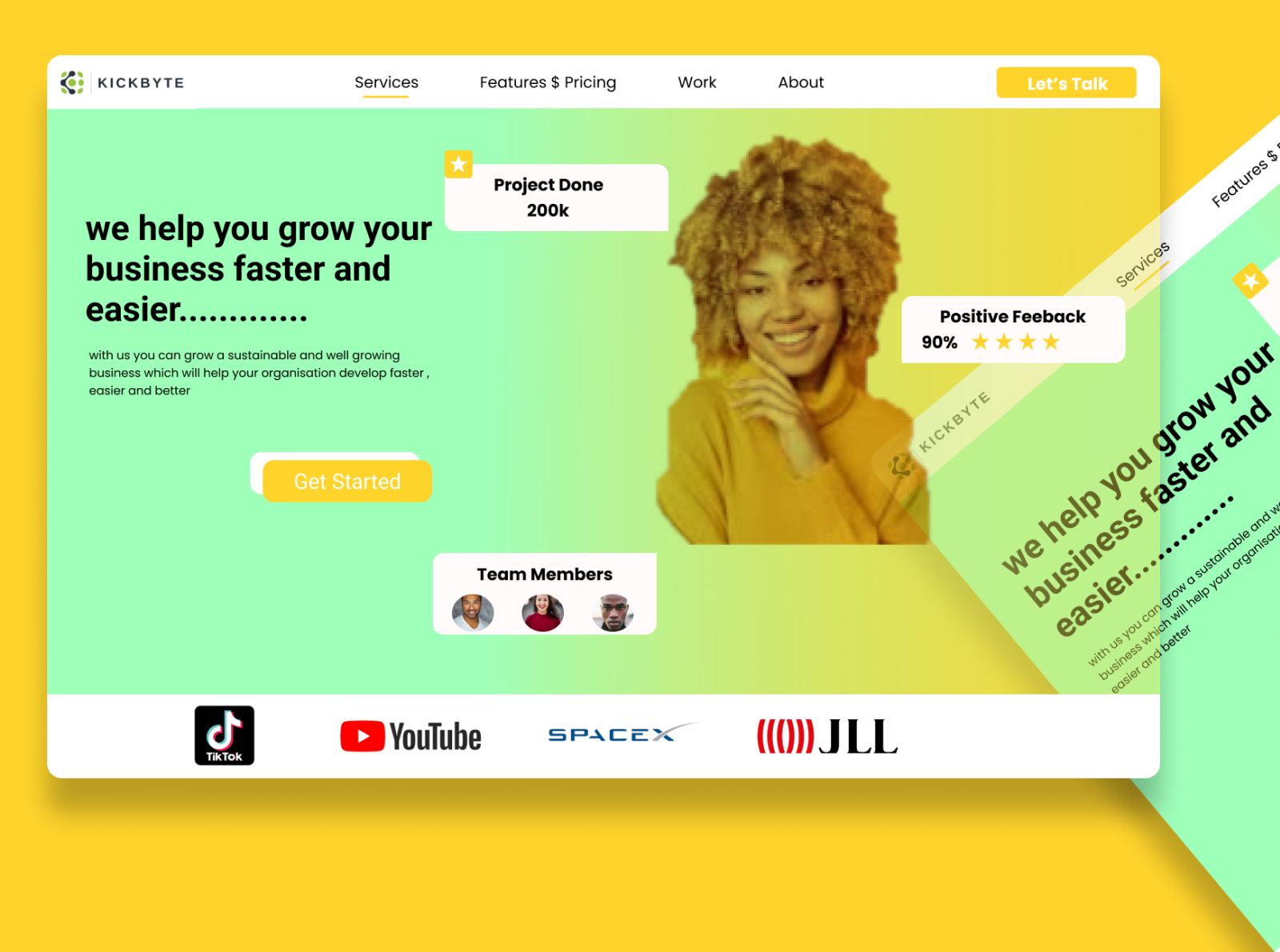The image presents a structured layout with a dark yellow background square as the overall frame. Inside this space, a larger, detailed square takes center stage.

At the top of this inner square, there's a white band, dividing the header. To the left side in this band, the brand name "KICKBITE" is prominently displayed in uppercase letters, with the unique spelling, K-I-C-K-B-Y-T-E. On the right side, the word "SERVICES" is underlined in yellow, followed by a series of navigation options including "FEATURES AND PRICING," "WORK," and "ABOUT."

Inside a yellow rectangle at the top right, there is a call-to-action in white text that says "LET'S TALK." Below this header area is an image of a smiling woman wearing a yellow sweater, posed with her hand thoughtfully under her chin. Adjacent to her image, in a white rectangle, there's a label that reads "POSITIVE FEEDBACK" with a rating of "90%" accompanied by four stars.

In the upper left corner of the woman's section, the text highlights "PROJECT DONE" with a notable figure of "200K" and beside it, a yellow square containing a star icon. To the left, in black text against the yellow background, there's a motivational message: "WE HELP YOU GROW YOUR BUSINESS FASTER AND EASIER."

Below this, another yellow rectangle displays another call-to-action with "GET STARTED" in white text. In the bottom right area, a white rectangle titled "TEAM MEMBERS" features three circles, each containing the image of a different person. The individual in the center of these circles is wearing a red sweater and is also smiling, contributing to the overall positive and inviting aesthetic of the entire layout.